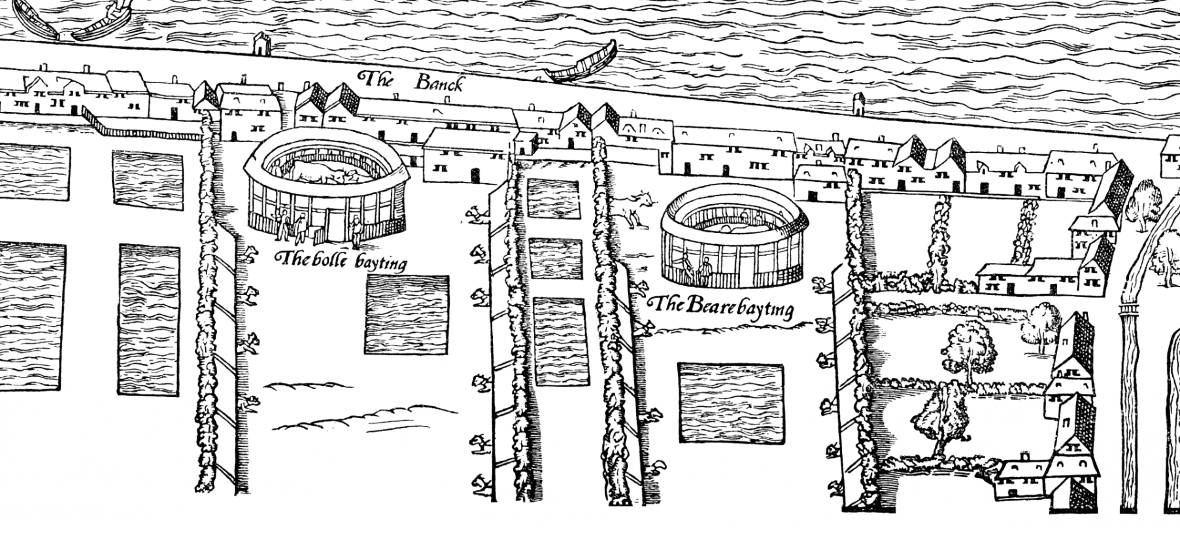This black and white pen-and-ink diagram, reminiscent of an old map, appears to depict a historical town or village, possibly from the Elizabethan period. In the top section, there's an expanse of water indicated by squiggly lines, with a few tiny, sail-less boats floating on it. Adjacent to the water is a label that reads "the Banc," spelled B-A-N-C-K. Below this label, a line of various-sized houses extends horizontally across the image. To the left side of the map, there are plots that appear to be gardens or farmland, bordered by periodic lines and squiggles, and possibly separated by trees or fences. Additionally, there are two circular arenas on either side of the middle section. The left arena is labeled "the Bull Baiting," suggesting activities like bullfighting, while the right arena, labeled "the Bear Baiting," is similarly surrounded by animals, indicating bear baiting events. Scattered around the arenas are more houses, vegetation, and trees, with a few buildings and trees visible towards the far right edge of the map.